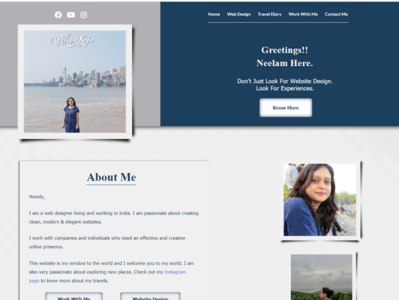The image seems to be a detailed promotional card or digital flyer. On a grey background in the upper left corner, the logos of Facebook, YouTube, and Instagram are displayed in white. At the center, mimicking a Polaroid format, there is an image of a woman standing near an ocean or lake with a large cityscape in the background.

The right side of the image features a deep blue background with white text at the top, although the specifics of the text are unreadable. Below this text is a prominent message, "Greetings to Exhibition Place. Noem here. Don't just look for website design, look for experiences," followed by a white button labeled "no more."

In the bottom left corner, the text "about me" is shown with an accompanying passage written in black, though the contents are unclear. Next to this section, on the right-hand side, is another digitally edited image designed to resemble a Polaroid. This picture features the same woman, darker complexion with black hair, wearing a blue shirt and glancing over her shoulder towards the camera. Below this, there's a final image depicting very dark, cloudy skies, again styled to look like a Polaroid photograph.